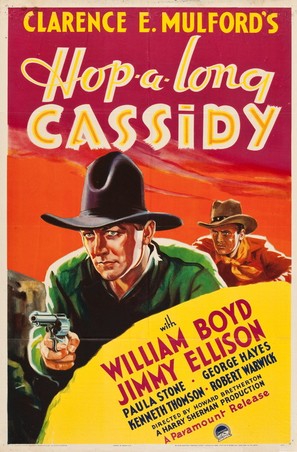This detailed vintage poster for the movie "Hopalong Cassidy" prominently features the title "Clarence E. Mulford's Hopalong Cassidy" in striking yellow and white cursive at the top. Below the title, two imposing cowboy figures dominate the scene against an evocative orange and red sunset sky. The foreground showcases a lawman or gunslinger wearing a black cowboy hat and an emerald green shirt, holding a silver revolver in his right hand aimed diagonally to the left. His expression is serious, with green eyes focused intently on a distant target. Positioned behind him, a slightly smaller and crouching figure, wearing a brown 10-gallon cowboy hat and an orange shirt with an orange scarf or ascot, looks forward, also with a stern expression. 

The rich, colorful sky enhances the dramatic tension of the scene, bathing both men in a warm, golden light that reflects off their clothes and faces. In the background to the right, a rock formation is faintly visible, adding to the rugged Western landscape. The bottom right corner features a yellow section where the names of the stars are listed: William Boyd and Jimmy Ellison in bold red lettering, followed by Paula Stone, George Hayes, Kenneth Thompson, and Robert Warwick in smaller black text. Further down, additional credits include "directed by Howard Bretherton, a Harry Sherman production, a Paramount release" along with the Paramount logo. The entire illustration brings to life the vintage, adventurous spirit of the era, perfectly capturing the essence of an old Western movie.